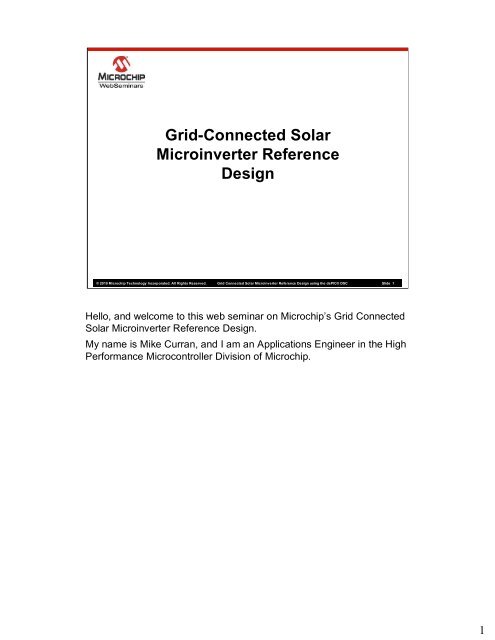**Caption:**

The image depicts a slide from a Microchip Web Seminar, predominantly featuring a white background with black text. At the top left corner, the title "MicroTrip Web Seminar" is visible. The main heading of the slide reads "Graded-to-Connected Solar Micro-Inverter Reference Design." Below the heading, the slide includes an introductory note, "Hello and Welcome to this Web Seminar on Microchip Graded-to-Connected Solar Micro-Inverter Reference Design. My name is Mike Curran. I'm an Applications Engineer in the High Performance Microcontroller Division of Microchip." Additionally, there is a small black banner at the bottom with illegible white text, presumably containing copyright or other formal information. The slide likely serves as an introduction to a technical presentation on solar micro-inverters, which are devices that convert DC from solar panels to AC for grid connectivity.